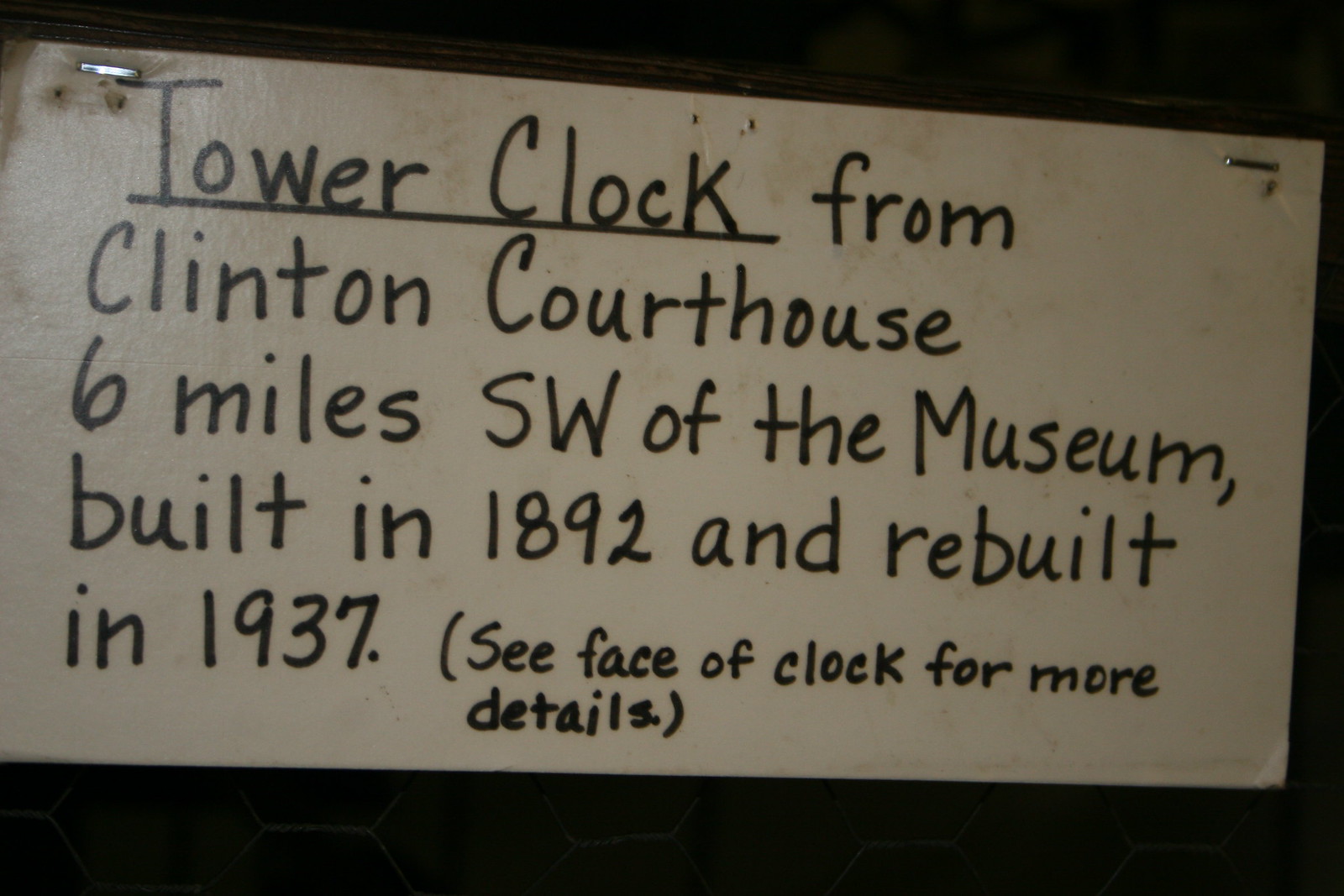This detailed rectangular photograph depicts a handwritten sign on slightly smudged white paper, illuminated from the left or upper-left side. The photograph has shorter left and right sides compared to its top and bottom, and the image is positioned mostly horizontally with a slight diagonal slant, lower side on the right. The background is dark, obscuring complete clarity, but it appears to include large, indistinct green soccer ball patterns or letters—possibly a “B” or an “8”—both too large to be fully captured within the frame.

The sign is stapled in the upper and left-hand corners, though the left staple protrudes slightly, and there are visible staple holes beneath it, suggesting the sign has been removed and re-stapled. The text on the sign is written in a mix of upper and lower case letters using what seems to be a black marker or thin Sharpie. At the top left, it reads “Tower Clock,” underlined with capitalized “T” and “C,” followed by “from Clinton Courthouse,” where “Clinton Courthouse” is also capitalized. The next line reads, “six miles southwest of the museum,” with “M” capitalized. The following lines state, “built in 1892 and rebuilt in 1937. (See face of clock for more details),” the latter in mostly lowercase except for the capital “S” of “See.” Given its casual presentation and context, the sign appears to be an informal small-town guide for a historical site, possibly relevant even into the year 2024.